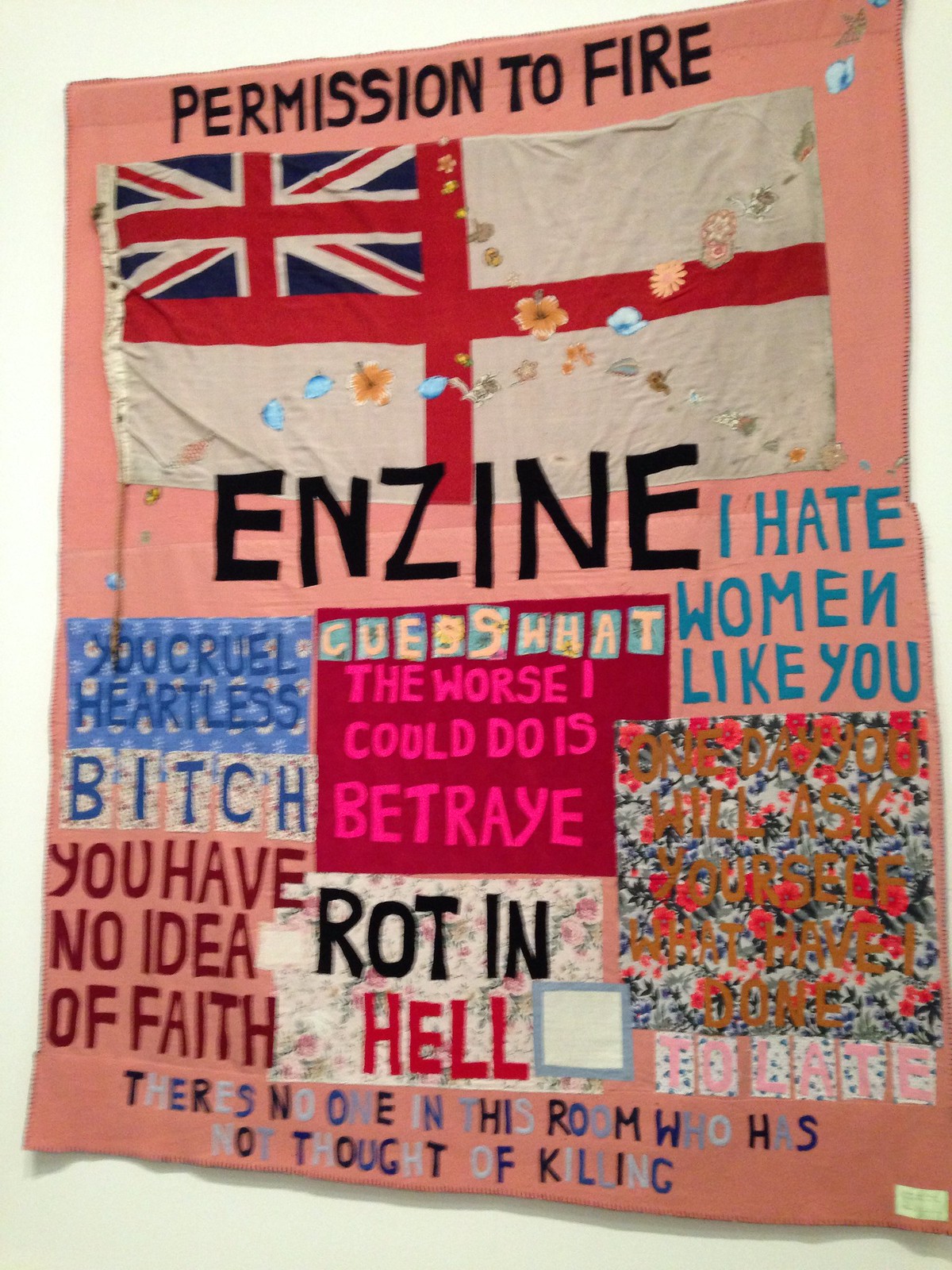This photograph features a large rectangular quilt-like fabric with a predominantly pink background, hanging on a white wall. The quilt, which has various pieces of fabric sewn onto it, includes prominently large black capital letters at the top reading "PERMISSION TO FIRE." Below this, in the center of the quilt, large black capital letters spell "ENZINE." The letters in this section are detailed with a peculiar artistic flair, such as a backwards "N" in the word "women." 

To the right, bold turquoise letters declare, "I HATE WOMEN LIKE YOU."

Beneath this, a series of phrases are sewn in different colors and fonts. One colorful patch reads "TOO LATE," while next to it, a red patch states, "THE WORST I COULD DO IS BETRAY." Near this is the word "BITCH" in pink lettering. Other notable phrases include "ROT IN HELL" and "YOU CRUEL HEARTLESS BITCH, YOU HAVE NO IDEA OF FAITH" found on different sections of the quilt.

In the top left-hand corner of the quilt, a white flag with red stripes and a British Flag in the left-hand corner is visible, adding a vivid nationalist flair to the chaotic composition.

Additional fabric sections reveal further messages in alternating colors, such as, "ONE DAY YOU WILL ASK YOURSELF WHAT HAVE I DONE?". At the bottom, creatively cut out letters spell out, "THERE'S NO ONE IN THIS ROOM WHO HAS NOT THOUGHT OF KILLING."

Overall, the quilt is a visually striking collage of colorful patches, bold statements, and eclectic fonts, evoking a sense of anger and betrayal expressed through textile art.